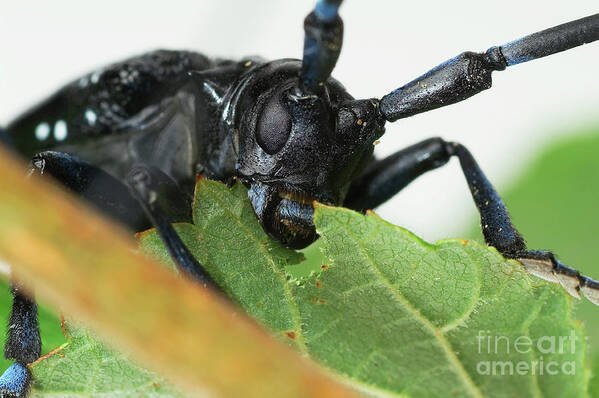The photograph is an extreme close-up view of a black beetle-like insect, highly detailed, and placed predominantly in the upper part of the image. The insect is in the process of eating a green leaf with brown-tipped edges and light green veins. Its large black eyes are positioned on either side of its head, with two large mandibles currently chewing on the leaf. The beetle's body and legs are black with small black hairs, while the lower sections of its feet are white. The segmented legs bend at the joints, holding onto the edge of the leaf. Two long antennae extend off the top of the beetle's head, with one pointing towards the top center and the other to the top right of the image, both partly extending off-screen. The beetle's semi-glossy black back catches the light subtly, revealing hints of blue highlights around its mouthparts, antennae, legs, and feet. The background is a soft, out-of-focus white, enhancing the detailed texture and color contrast of the beetle and the leaf. A beige twig intersects diagonally from the left to the bottom center of the image, adding depth. At the bottom right corner, the photograph is watermarked with "Fine Art America" in a slightly transparent font. The image exemplifies photographic representational realism.